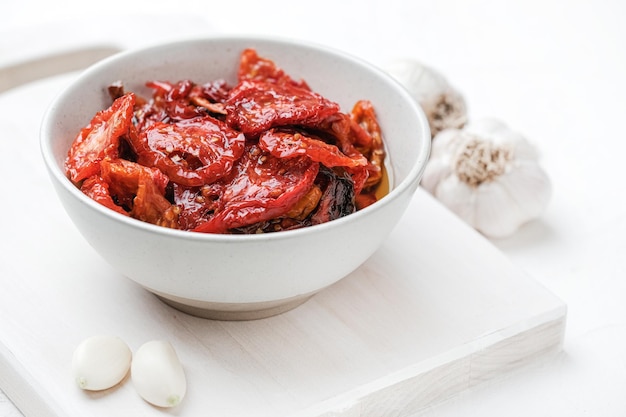This photograph prominently features a white bowl filled with sun-dried tomatoes in various shades of red, orange, and brown. The bowl is situated on a white cutting board that has the appearance of wood, adding a rustic touch to the composition. Positioned to the left of the bowl, there are two peeled garlic cloves, while to the right of the cutting board rest two whole heads of garlic. The bowl itself is illuminated by a bright, focused light that creates a sharp reflection on its surface, further drawing attention to the colorful tomato pieces stacked inside. The background includes a hint of a white chair, adding depth to the setting. The overall image is slightly blurred, suggesting a professional artistic intent, with a clear emphasis on the culinary elements.